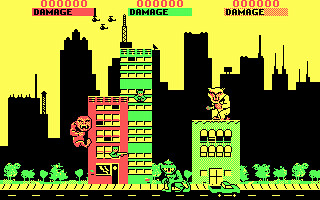This detailed screenshot from the classic 1980s video game "Rampage" depicts a rudimentary cityscape dominated by three primary buildings. To the left is a boxy red building with yellow windows, which features a gorilla climbing its facade, likely a character inspired by King Kong. A green man with a gun is visible leaning out of one of the windows, aiming at a lizard monster situated on the road below. Adjacent to the red building is a slightly taller light green building. To the right stands the shortest of the trio, a green building with yellow windows, atop which a wolf-like boss character menacingly oversees the chaos. Between the buildings and street level is a yellow line representing the pavement, outlined with scattered trees. A small green car is visible on the road, pursued by the aforementioned lizard monster. In the background, a silhouetted metropolitan skyline under a yellow sky sets a dramatic backdrop, accompanied by three black helicopters hovering in the distance. At the top of the screen, red, green, and pink bars display "damage" levels, all currently set at zero, likely indicating the health status of various characters within the game. This portrayal encapsulates the basic yet captivating graphics characteristic of early NES systems, bringing nostalgic memories of monster mayhem and building destruction à la "Rampage."